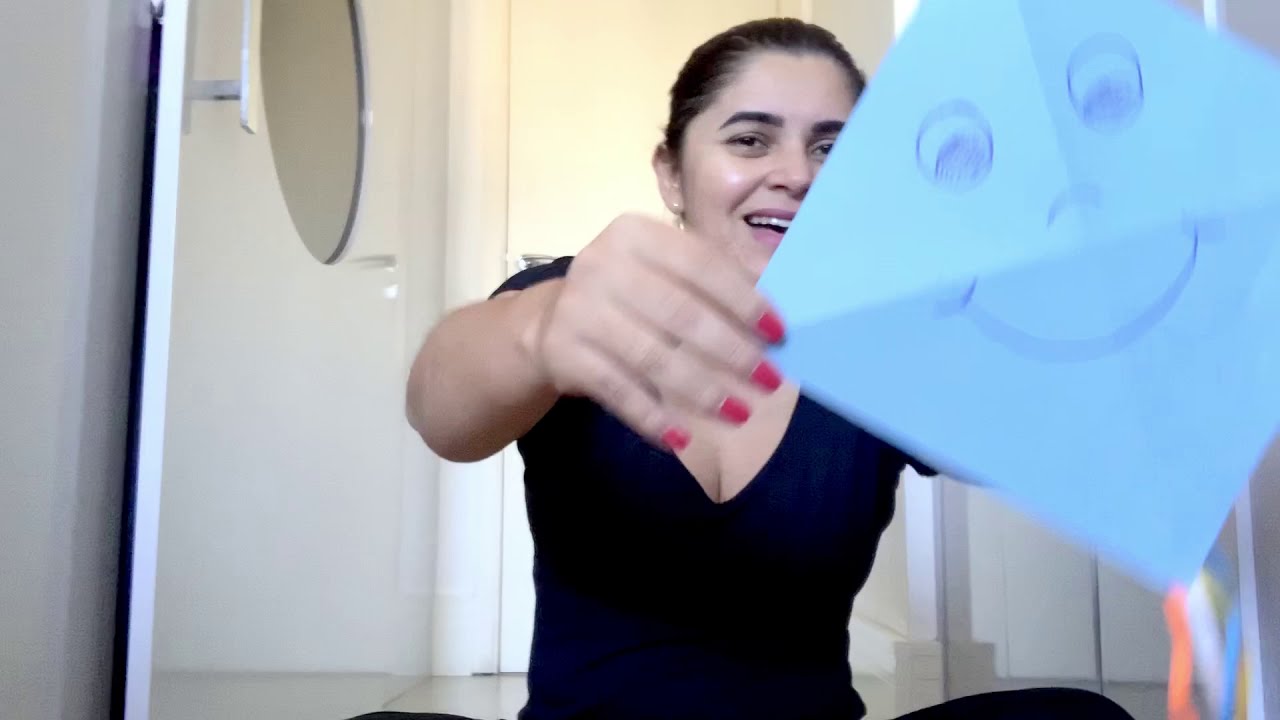In this indoor photograph, a young woman with fair skin and slicked-back black hair sits cross-legged on the floor. She’s wearing a black v-neck shirt and smiling softly, her mouth open in a half-smile. The image captures her from the waist up, with her hands extended forward, holding a light blue square piece of paper that is folded into quarters. The paper features a hand-drawn smiley face, with one eye on each quarter and a curved arch for a nose, accompanied by a smile at the lower half. Her nails are painted pink, and she wears a stud earring. The room's background is predominantly white, with a circular window or mirror on the left and another white wall behind her. Additionally, some yellow or orange streamers hang from the bottom of the blue paper she holds.